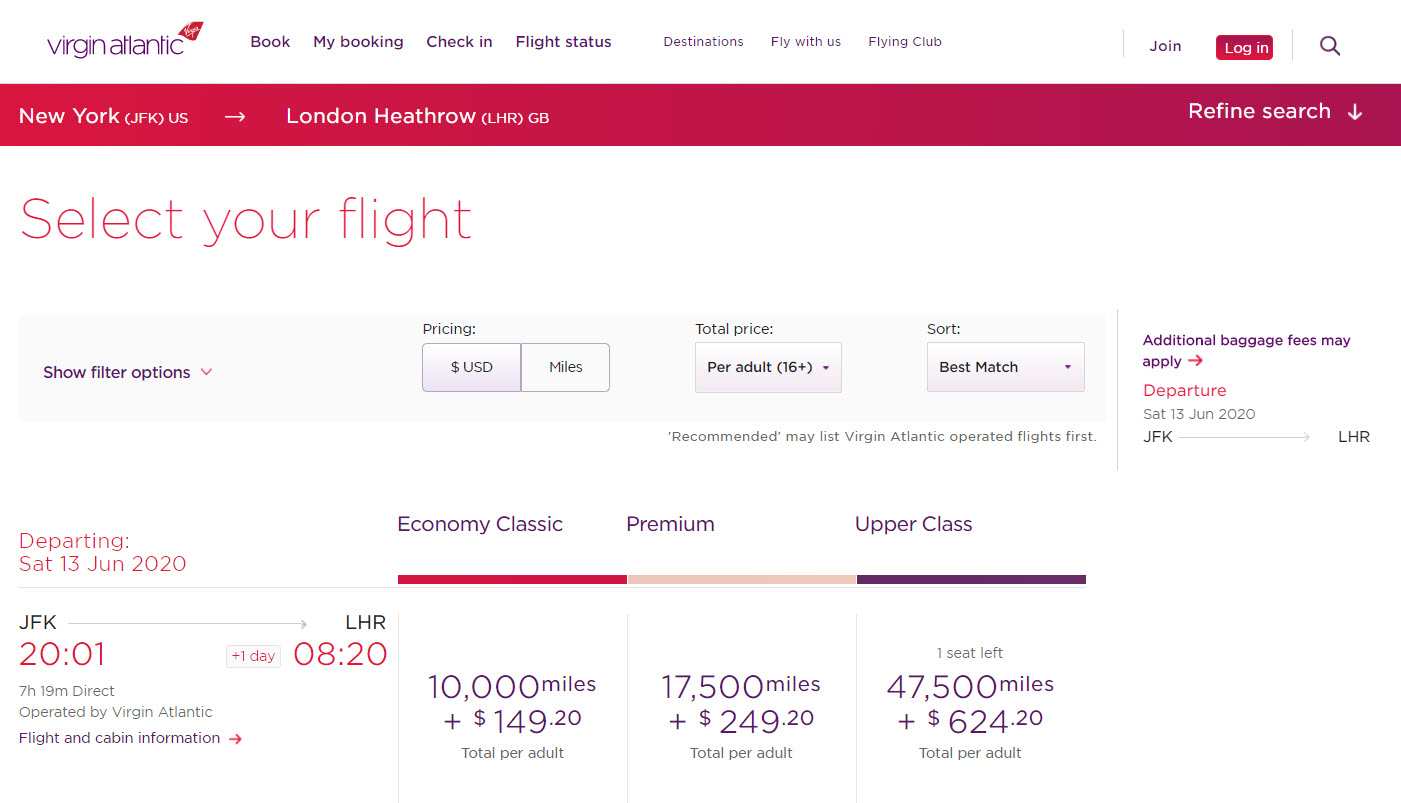A detailed and clean caption for the described image is:

"This image displays an active web page for booking flights on the Virgin Atlantic airline website. The web page has a landscape orientation and features several navigation options at the top including 'Booking', 'My Booking', 'Check-In', 'Flight Status', and options for logging in or joining. The user is searching for a flight from New York's JFK Airport to London Heathrow Airport (LHR). They have set filters for displaying prices in United States dollars, total price per adult, and sorting results by the best match. The selected flight is a direct flight lasting 7 hours and 15 minutes. The webpage shows different fare options: Economy Classic for 10,000 miles plus $1.50, Premium for 17,000 miles plus $250, and Upper Class for 47,500 miles plus $625. The user appears to be utilizing their accumulated mileage to purchase the flight."